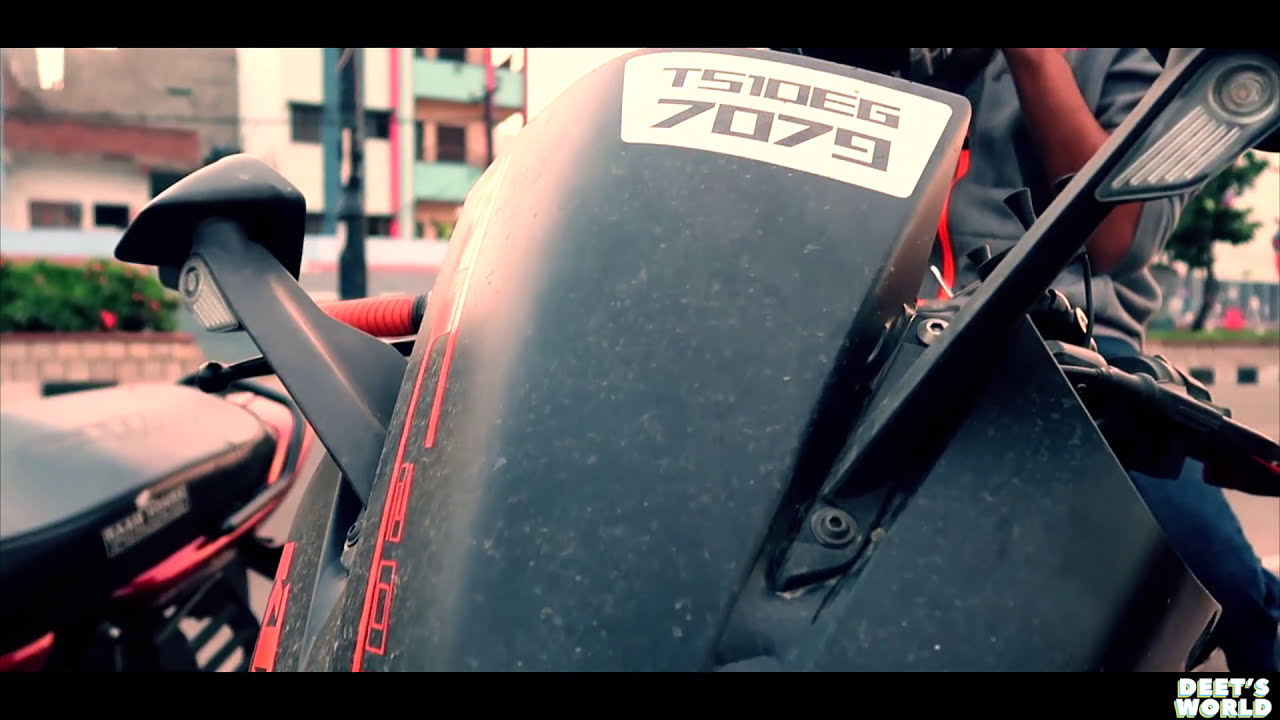The image is an extremely close-up view of the front of a black motorcycle with red detailing. Prominently displayed on the top portion of the motorcycle’s windshield is a white trapezoid with the text "T510EG" above "7079." To the upper right of the motorcycle front, parts of a person wearing a gray or blue shirt and jeans are visible, though the rest of the person's body is cut off. The background is out of focus but shows what appears to be older buildings. One is a tan-colored, two-story building with mint green balconies adjacent to a light pink building. To the bottom right of the image, the text "Dietz World" is visible in white letters. Additional features include two lights protruding from the sides of the motorcycle and possible presence of another black motorcycle with red trimming to the left.